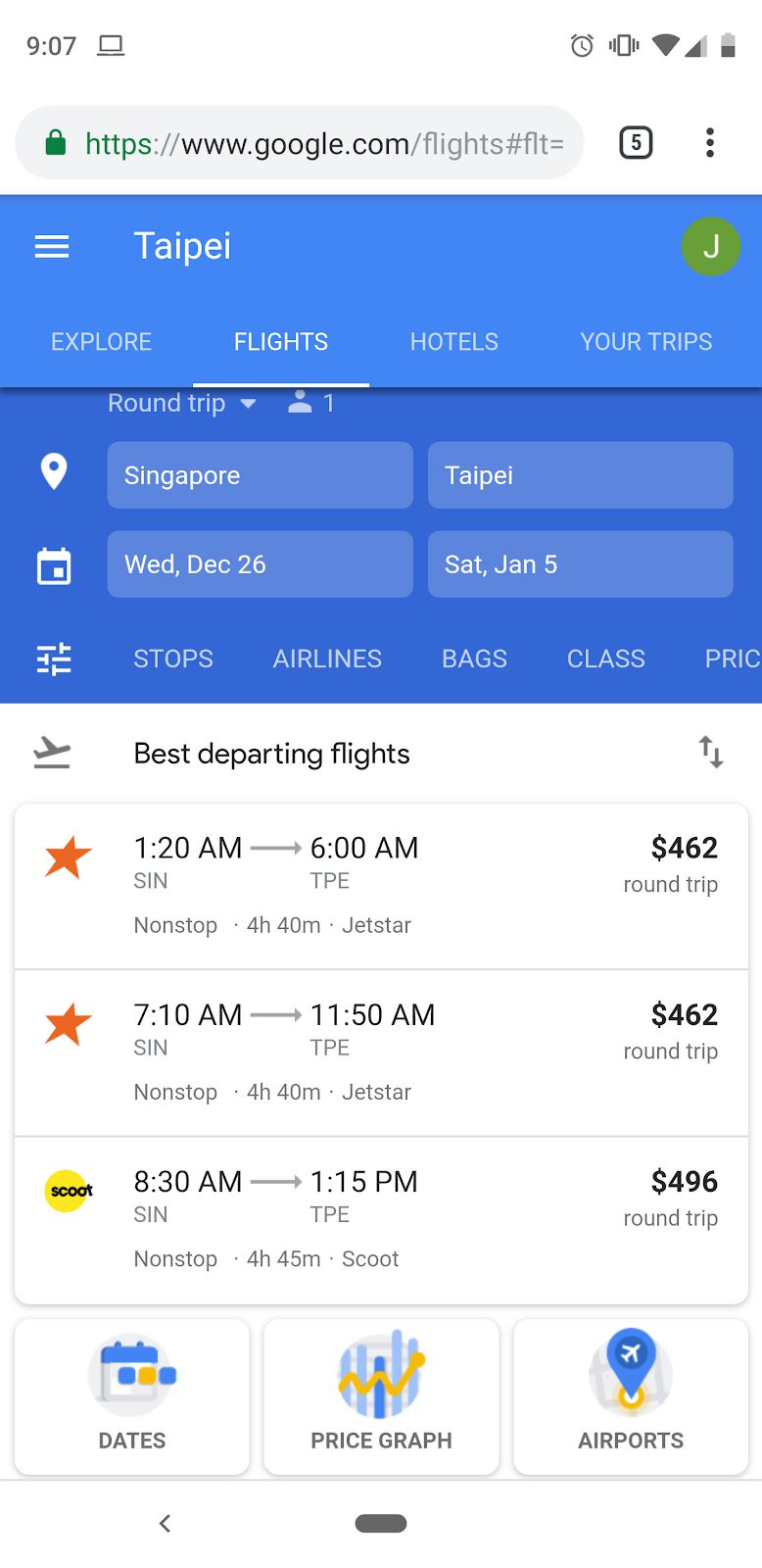The image displays a mobile screenshot of the Google Flights website, captured at 9:07 AM, as indicated by the time in the upper-left corner of the white status bar. In the upper-right corner, various icons show an alarm, vibrate mode, Wi-Fi signal, and a half-full battery.

The URL bar shows "https://www.google.com/flights," alongside icons for five open tabs and a three-vertical-dot menu for more options. Below the URL bar, a blue header features the word "Taipei" in white text next to three horizontal lines. 

The website section prominently showcases the "Explore Flights, Hotels, and Your Trips" menu with the "Flights" tab highlighted. Adjacent to these options, a green circular icon with the letter "J" in white stands out.

The search criteria detail a round-trip flight from Singapore to Taipei, scheduled from Wednesday, December 26th to Saturday, January 5th. Below this, filter options for stops, airlines, baggage, class, and price are available next to a filter icon.

Listed departing flights include the following:
1. Departs at 1:20 AM from SIN (Singapore Changi Airport) to TPE (Taipei Taoyuan Airport), priced at $462 for a round trip.
2. Departs at 7:10 AM from SIN to TPE, priced at $462 for a round trip.
3. Departs at 8:30 AM from SIN to TPE, priced at $496 for a round trip.

The screen also displays a date selector, a price graph, and an airport icon, providing additional context and interactive options for the user.